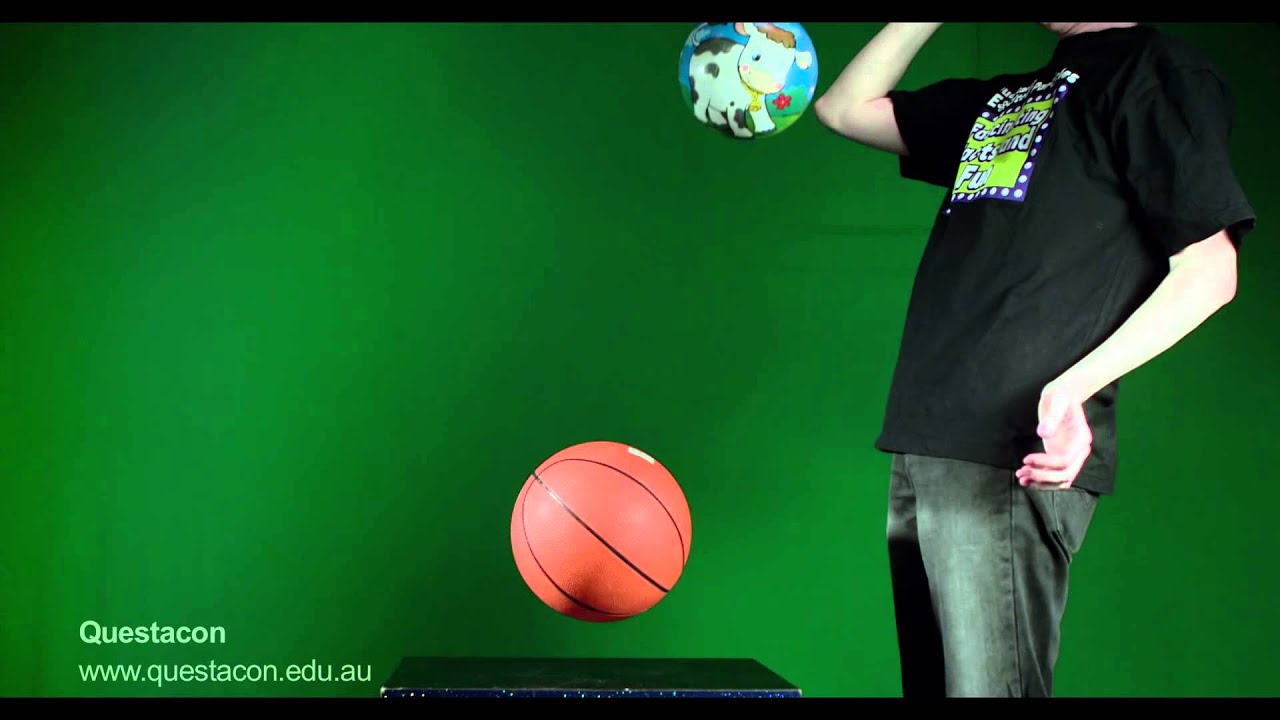In this highly detailed indoor photograph, a person with white skin is depicted from the neck down, standing on the right side of the frame. They are wearing a black t-shirt adorned with a fluorescent green and purple design, which appears to be some form of advertisement, though the crumpled shirt partially obscures the text. Their left arm is slightly bent at the elbow, resting by their side, while their right arm is raised with the elbow bent, touching a ball that features a cartoon cow image. The scene includes two bouncing balls: one orange basketball in midair, possibly rebounding off a small tabletop, and another higher ball showing the cartoon cow. The background is green, likely a green screen, with the text "Questacon www.questacon.edu.au" written in lighter green situated in the lower left corner of the image.